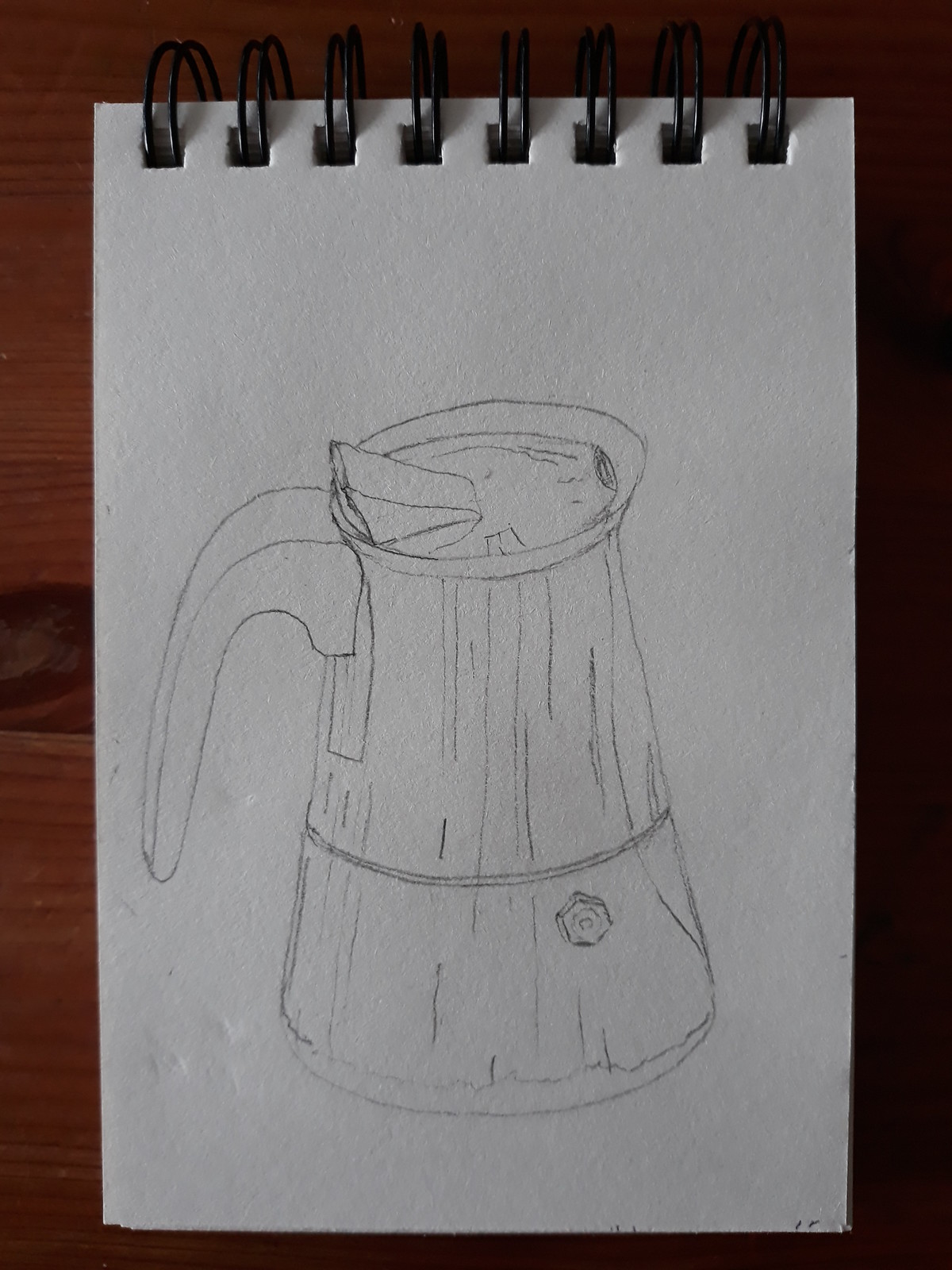This image showcases a portrait-style sketch pad with a black ring binder at the top, allowing the white sheets to be flipped from bottom to top. The pad is positioned on a dark brown wooden or faux wood table. The current sheet features a detailed pencil sketch of a jug or pitcher that appears to contain liquid, possibly a cocktail, given the inclusion of pencil blobs suggesting pieces of fruit floating inside. The rounded jug has a varying diameter, expanding from top to bottom, and includes a single handle on the left side. Additionally, there is a tab on top of the jug, which might be a spout cover, and a button on its front, enhancing its three-dimensional appearance. The shaded areas on the sketch suggest depth and contours, portraying a realistic view of the jug.